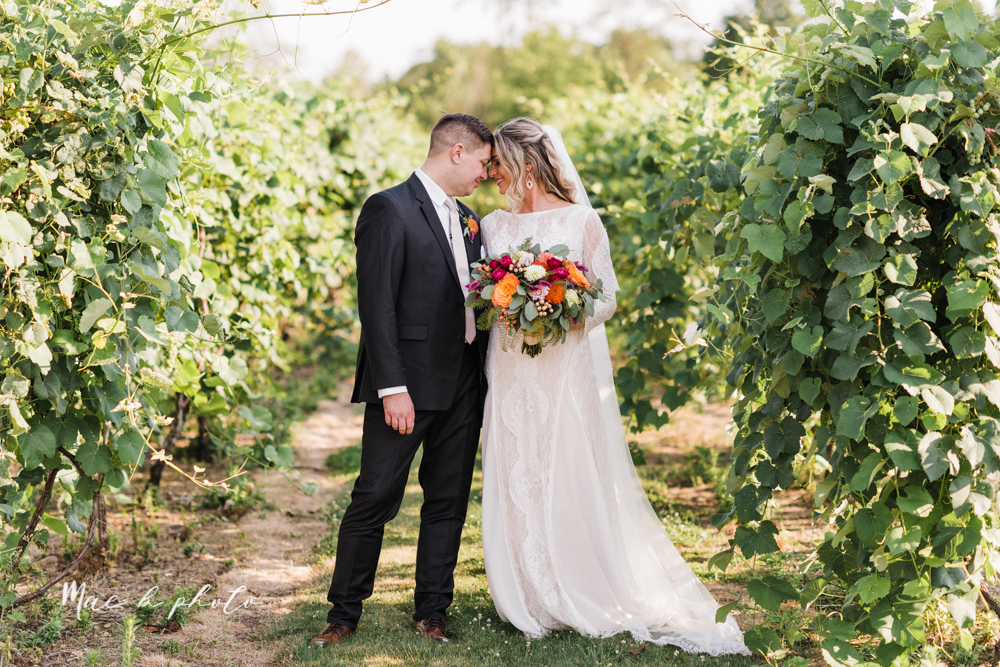In this captivating wedding photo, a newly married couple stands in a picturesque vineyard with lush grapevines and diverse green shrubs surrounding them. The bride, radiating joy with her blonde and brown hair, is adorned in a flowing white gown that elegantly drags on the ground. She holds a vibrant bouquet featuring magenta and white roses, complemented by striking orange blooms and verdant leaves. Beside her, the groom looks dapper in a black suit paired with a white collared shirt. Their foreheads gently touch in a tender, intimate moment, both basking in the bright, golden sunlight. The field behind them, filled with tall green plants and high foliage, adds to the serene and romantic atmosphere. In the bottom left corner of the image, the photographer's signature subtly marks this beautiful memory.